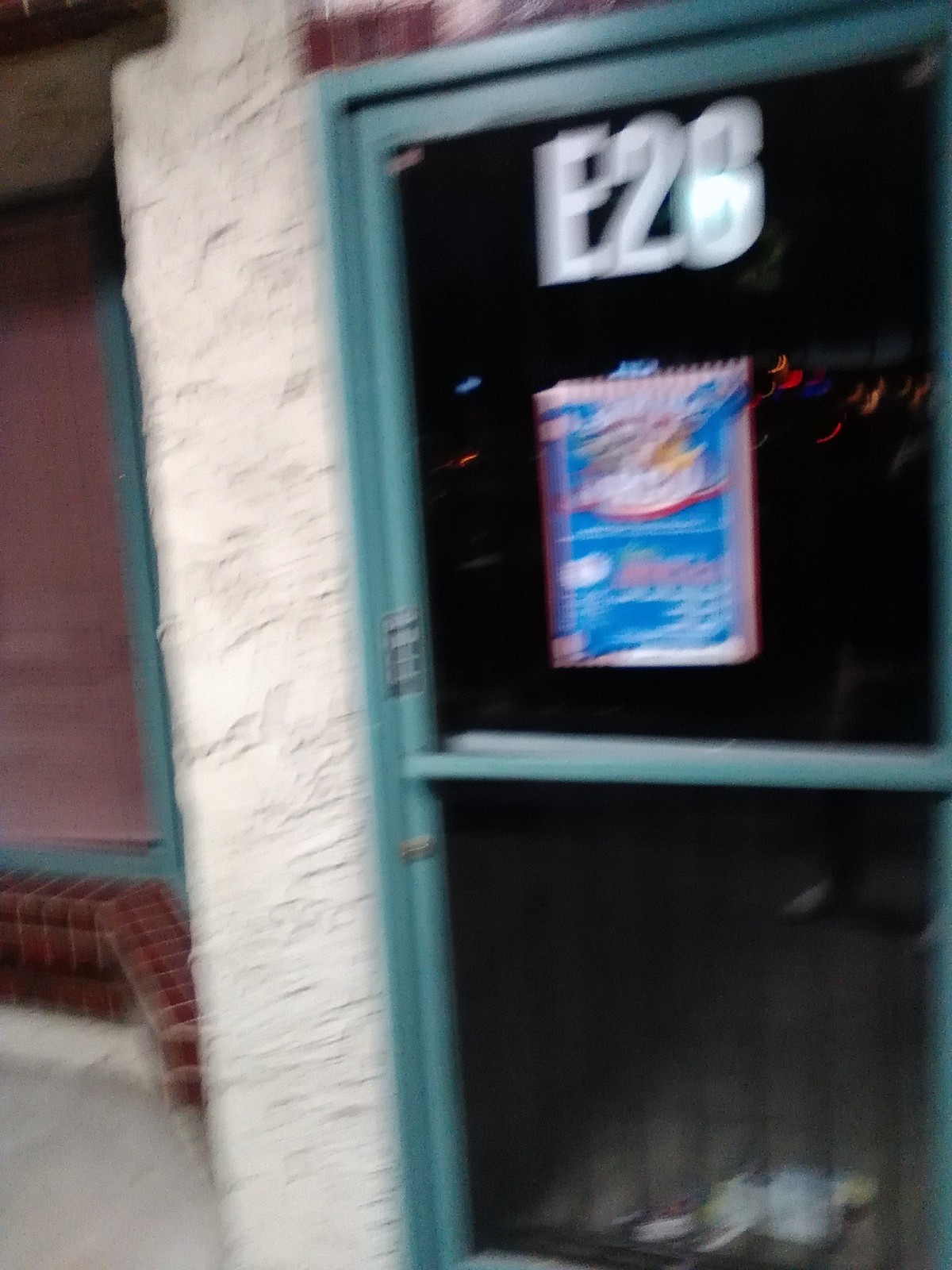This photograph captures the entrance to what appears to be a storefront or business establishment. The image is slightly blurry but features a glass door framed by a green metal outline. The door is equipped with a horizontal handle, clearly marked with the word "PULL" towards its center. Above the door, in white text, the identifier "E26" is prominently displayed. The surrounding area of the door is finished with a textured stucco surface, adding a rustic touch to the entrance.